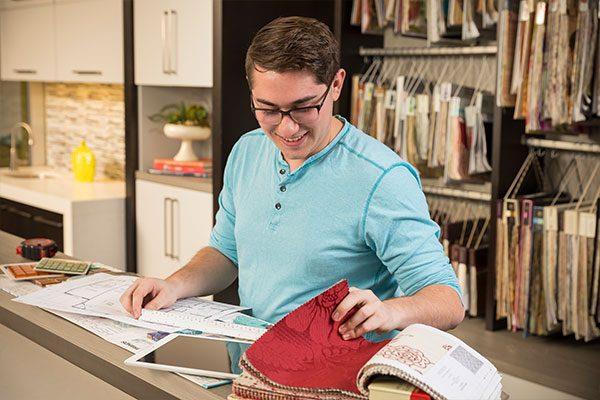In the photograph, a Caucasian man, sporting black-rimmed glasses and an aqua blue cardigan with sleeves rolled up to the elbows, stands at a light gray wooden counter. He is closely examining an open fabric sample book with a bright red floral page, smiling as he works. The counter before him is strewn with blueprints, some tile backsplash samples, a measuring tape, and a white-framed black-screened tablet. He has his right arm resting on the scattered papers while he focuses on the fabric designs. 

Behind him, the background reveals shelving with metal rods adorned with strings holding an assortment of pastel fabric samples. To the left, partially blurred, is a black partition leading to a demo kitchen area. This kitchen setup features white cabinets, both upper and lower, accented with a gray countertop. On the counter is a small houseplant in a white holder, a metal sink with a gracefully curving faucet, and a yellow vase prominently positioned next to the sink. This pristine demo display is likely used to illustrate potential kitchen designs to customers.